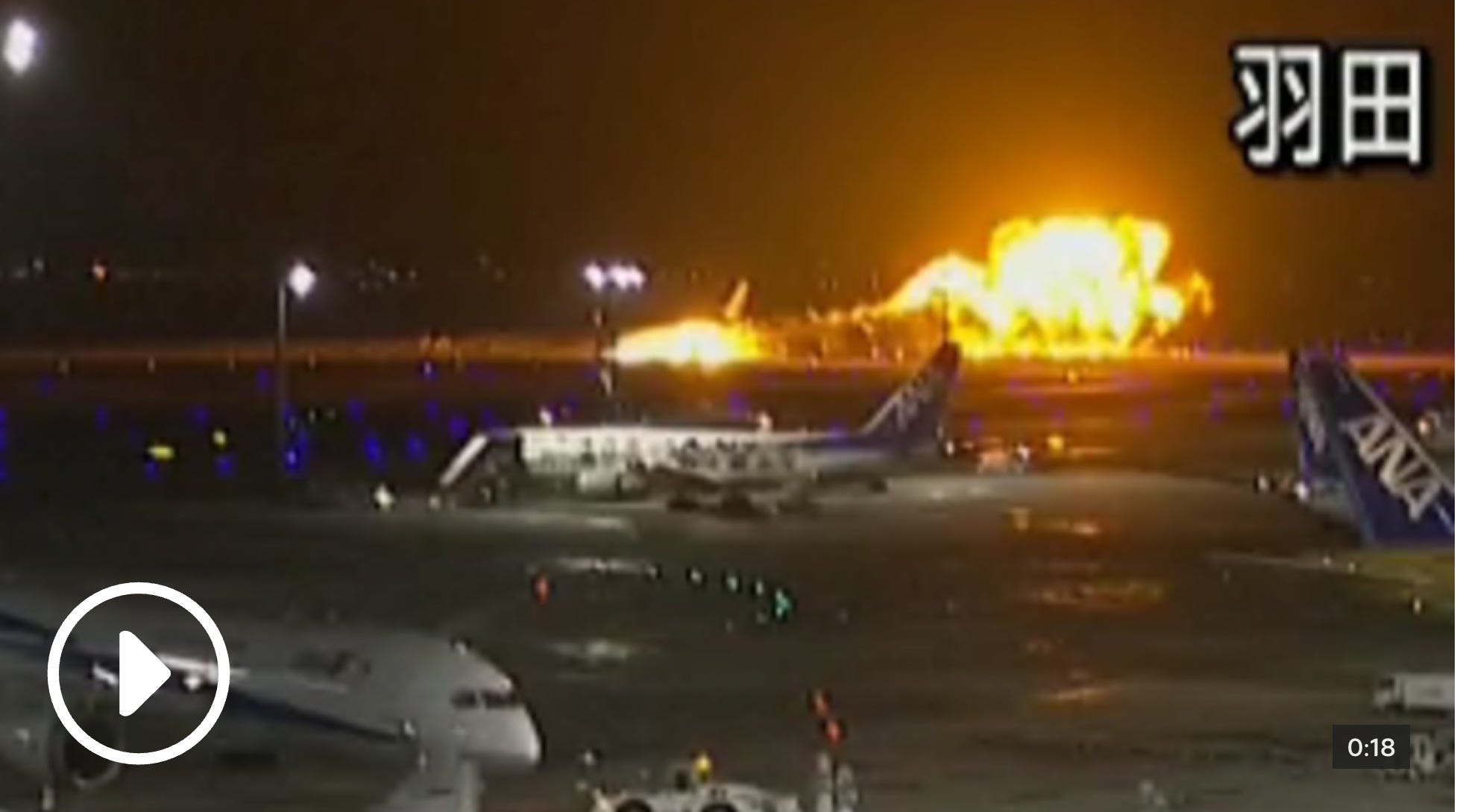The image is a paused video from what appears to be 1990s-era airport surveillance footage. The scene is set at night and captures an intense explosion in the background on a damp-looking runway. The foreground features three planes: a full airplane with the letters ANA on its blue tail, a half airplane, and just the tail of another plane. The main visible plane is white with blue accents. Surrounding the planes are small blue lights and two large floodlights near the middle plane. A luggage truck can be seen at the center. The video has a timestamp showing 0 minutes and 18 seconds, and there is a play button on the bottom left corner. Additionally, Chinese or Japanese characters are visible in the top right corner of the frame. The explosion is notably bright, with a white-orange glow and a trailing effect, suggesting a recent incident.